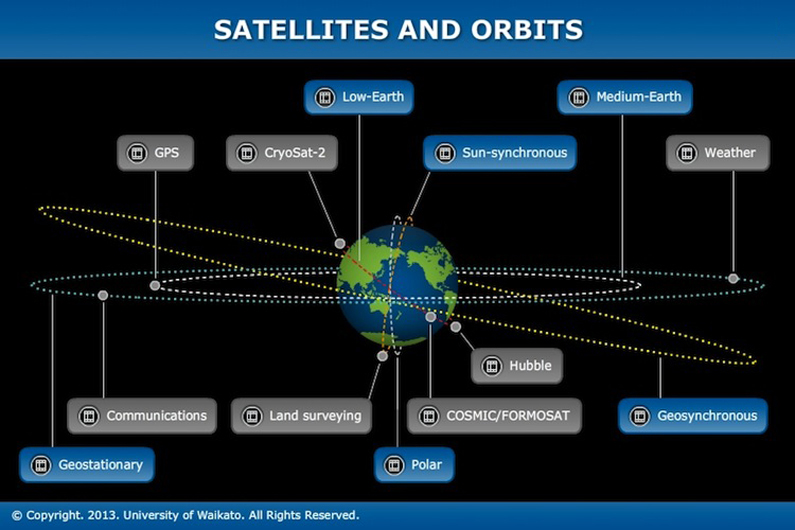This image, copyrighted in 2013 by the University of Waukota, features a detailed diagram of the Earth surrounded by various satellite orbits. At the top, the diagram begins by illustrating the orbits of different satellites, starting with GPS in white dotted lines. Moving towards the center, we see the orbits of CryoSat-2 in red dotted lines, followed by low Earth orbits and sun-synchronous orbits. Medium Earth orbits and weather satellites are depicted with green or blue dotted lines. Further down, the diagram highlights geostationary orbits, polar satellites, land surveying satellites, communications satellites, Cosmic Formosat, and the Hubble Space Telescope in geosynchronous orbit.

Each satellite orbit is depicted as a spiral or circular path around the Earth, clearly showing their respective positions and altitudes. The central globe, representing the Earth, is encircled by these varied orbits, demonstrating the complexity and diversity of satellite systems. The diagram comprehensively covers a wide range of satellite functions and orbit types, underscoring the vast number of satellites in operation.